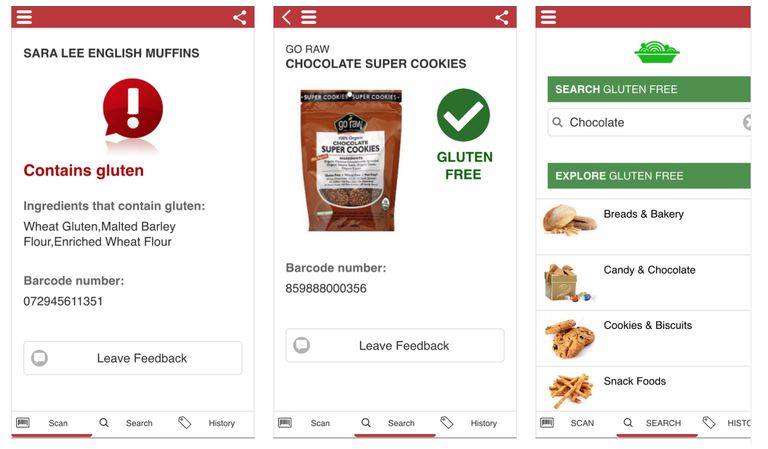The image features three distinct food presentations available for purchase, organized from left to right. 

On the left, a banner adorned with vivid red highlights showcases "Sara Lee English Muffins." A prominent red warning sign alerts consumers that the product contains gluten, specifying components such as wheat gluten, malted barley flour, and enriched wheat flour. The presentation also displays a barcode and an option for leaving feedback.

In the center, the focus shifts to "Go Raw Chocolate Super Cookies," highlighted as gluten-free with green text and a green checkmark. Similar to the first image, this listing includes a separate barcode and an option to provide feedback.

The third image on the right serves as a search interface for locating gluten-free products. It lists categories such as breads and bakery items, candy and chocolate, cookies and biscuits, and snack foods. Along the bottom of each section, various options are highlighted with red markers: "scan" for the first image on the left, and "search" for the central and right images, emphasizing their selected functions.